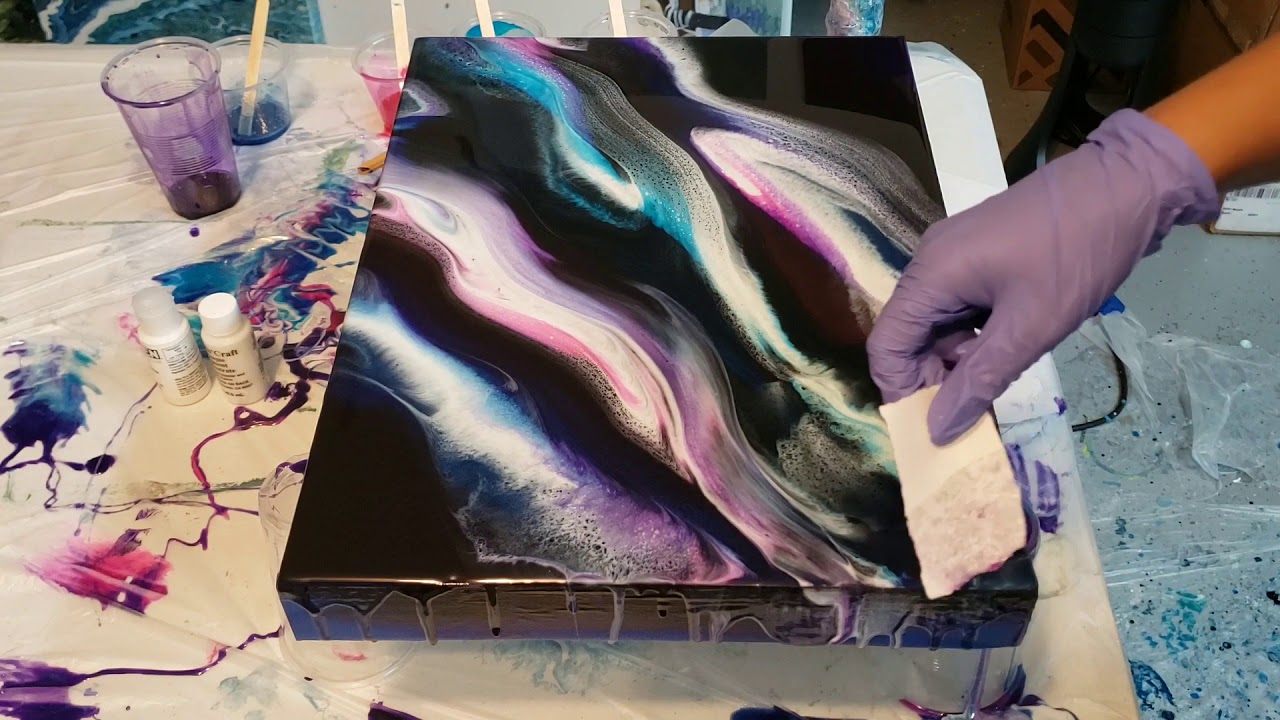This photograph captures an intricate and colorful art project in progress, resembling a fusion between traditional painting and hydro dipping techniques. Central to the image is a canvas coated in deep, glossy black paint, creating a striking backdrop. Vivid white, pink, and various shades of blue and purple paint have been dynamically splashed and streaked across the surface, from the upper left to the lower right, forming a vibrant, almost gradient-like pattern. In the lower right-hand side of the photo, a light brown-skinned man, donned in a purple latex glove, uses a white block or sponge to manipulate the paint, adding fluidity and texture to the artwork. The canvas rests on a table protected by a plastic sheet, surrounded by a slightly messy array of mixing cups and painting materials, hinting at the custom blending of colors used in this creative process. The protective plastic extends to the floor, ensuring a clean workspace amidst the artistic endeavor.